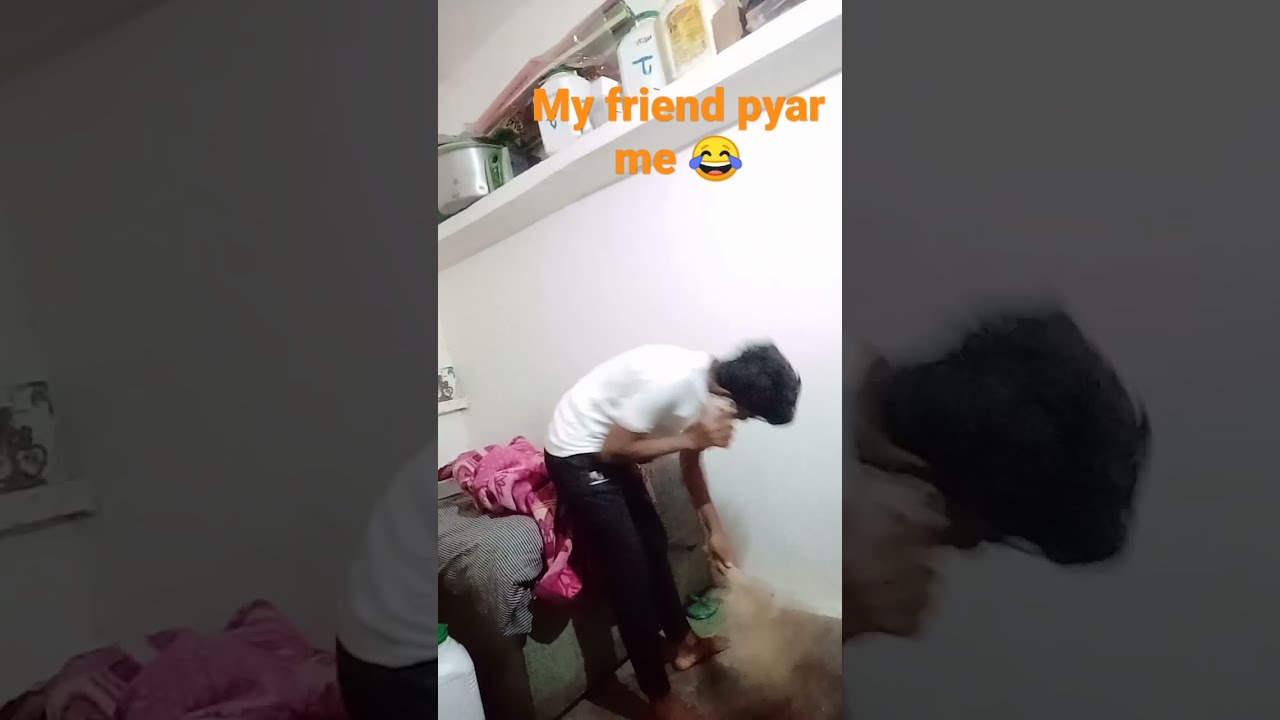In a poorly quality photograph taken in a bedroom, a person with black hair, wearing black pants and a short-sleeved white t-shirt, is seen bent over at the foot of an unmade bed that features a pink blanket. The individual is engaged on their phone using their right hand while their left hand appears to be interacting with something blurred in the foreground, possibly a pet or an object. Above them, a white wall-mounted shelf loaded with large containers, including jugs, barrels, and possibly a pressure cooker, looms somewhat precariously. The scene is also layered with a zoomed-out, filtered background and adorned with orange text that reads "my friend, Pyar, me," followed by a laugh emoji. This crowded composition suggests a casual yet cluttered personal space.